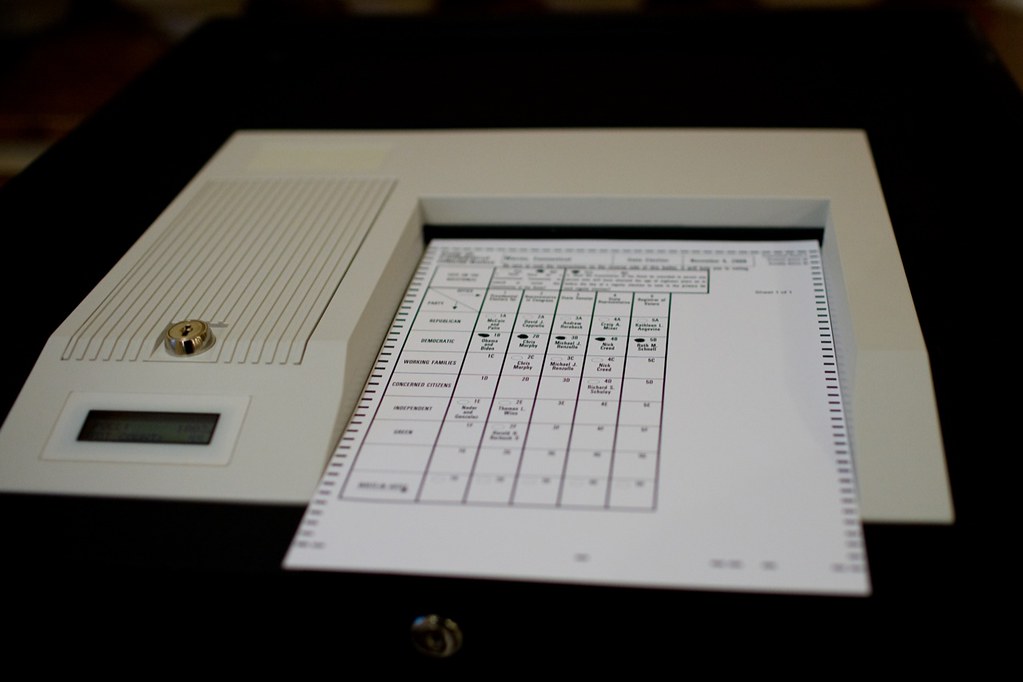The image features a piece of office equipment that resembles a register or printer, situated in a dimly lit room. The machine is square-shaped with a cream-colored top and a black bottom. A gold-colored keyhole is discernible on a ridged flap at the top, which likely serves as a lockable compartment. Below this keyhole, a small digital display screen shows numerical data, possibly the page count. The left side of the machine has an indented design. On the right side, there is a paper slot where a white sheet of paper, featuring a grid-like chart with columns of numbers and words, is visible. The sheet has perforated edges, suggesting that it can be torn off into sections.